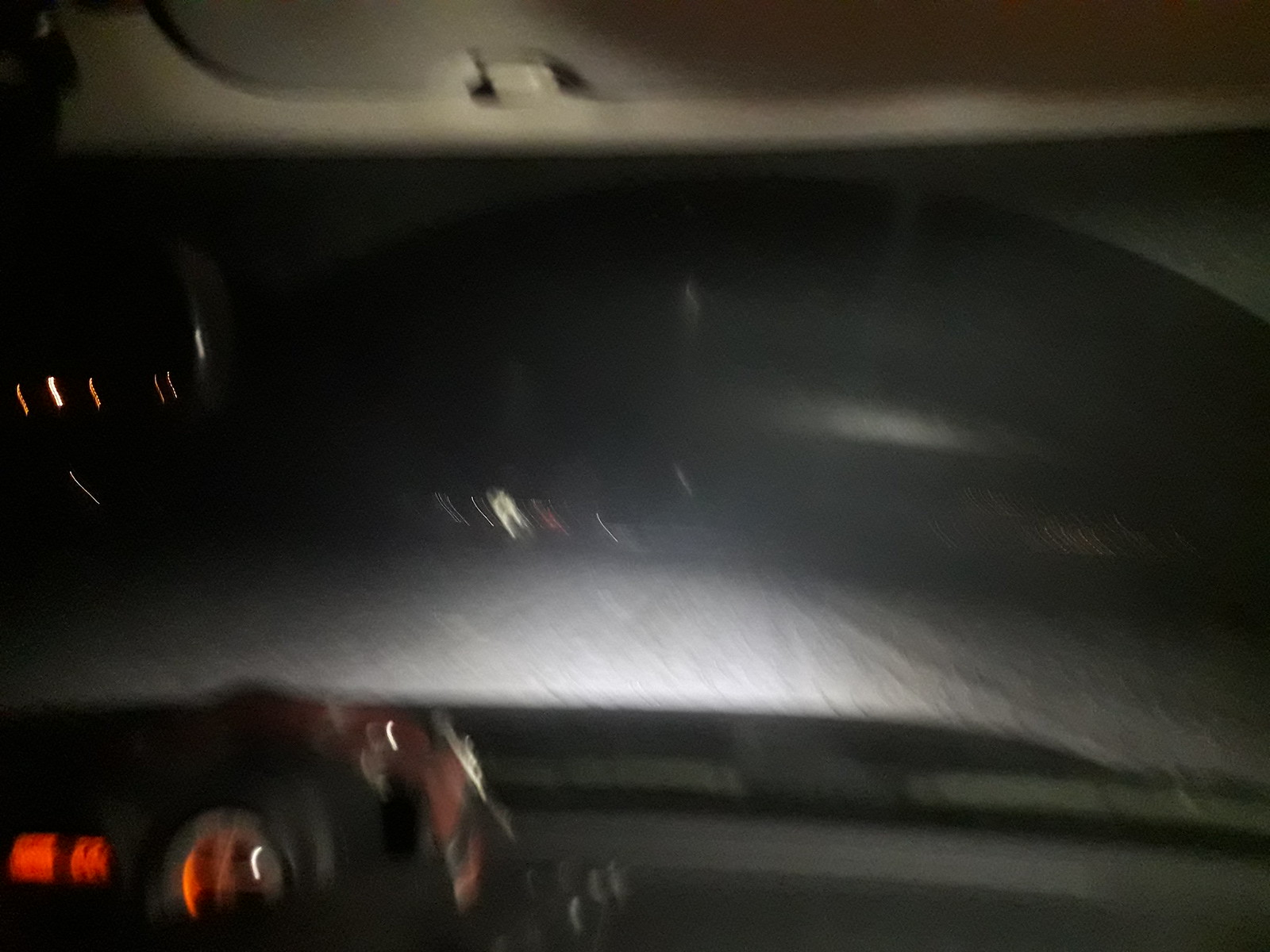The image is a blurry nighttime photograph taken from the passenger side of a vehicle. The darkened interior reveals the dashboard illuminated by orange lights, casting a glow across various dials and controls. The windshield frames the view ahead, where the road, partially illuminated by the vehicle's headlights, appears white, possibly due to snow, though the low shutter speed makes it difficult to be certain. Streaks of blurred white and orange lights from distant sources punctuate the otherwise dark environment, suggesting motion. The top of the image features a tan strip running horizontally, and there's a hint of the vehicle's maroon and black steering wheel in the bottom left-hand corner, adding to the overall sense of being inside the car.